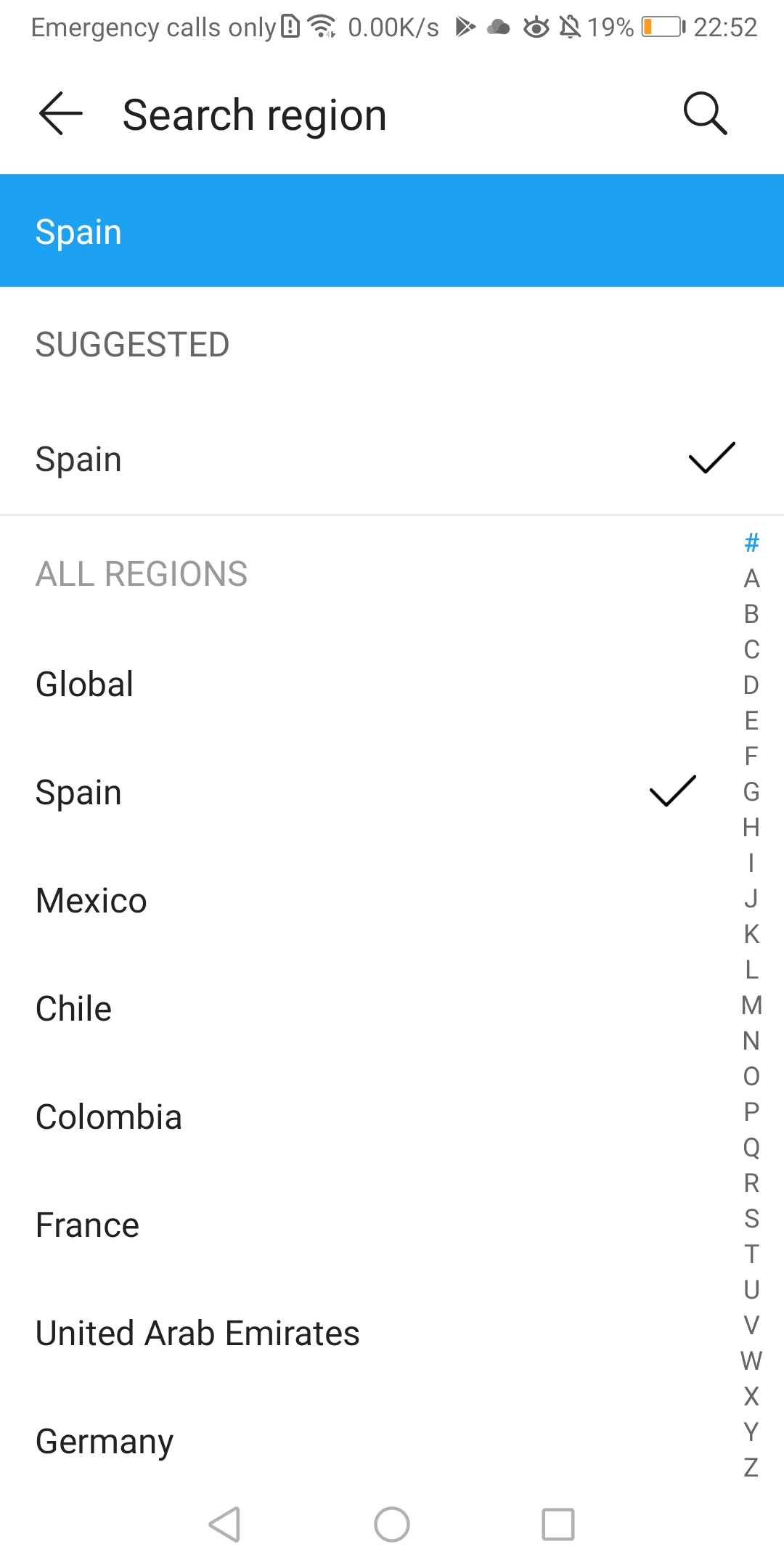This image depicts the screen of a cell phone. At the top, the notification bar indicates "Emergency Calls Only" beside icons that show no active wireless connection (0.00k/s), a muted notification bell, and a battery at 19% charge. The time displayed is 22:52. Below this bar is a back arrow labeled "Search Region" with a magnifying glass icon on the far right.

Underneath, a medium blue rectangle features the country name "SPAIN" in white text. Further down, "SUGGESTED" is in black, all-capitalized letters against a white background, with Spain listed again and marked with a checkmark on the right.

Scrolling further reveals a list of selectable regions: "Global," "Spain" (also checked), followed by "Mexico," "Chile," "Colombia," "France," "United Arab Emirates," and "Germany." The far right side of the screen sports an alphabetical index (A-Z) for easier navigation.

At the bottom of the page are navigation icons: a left-pointing arrow, a circle, and a square.